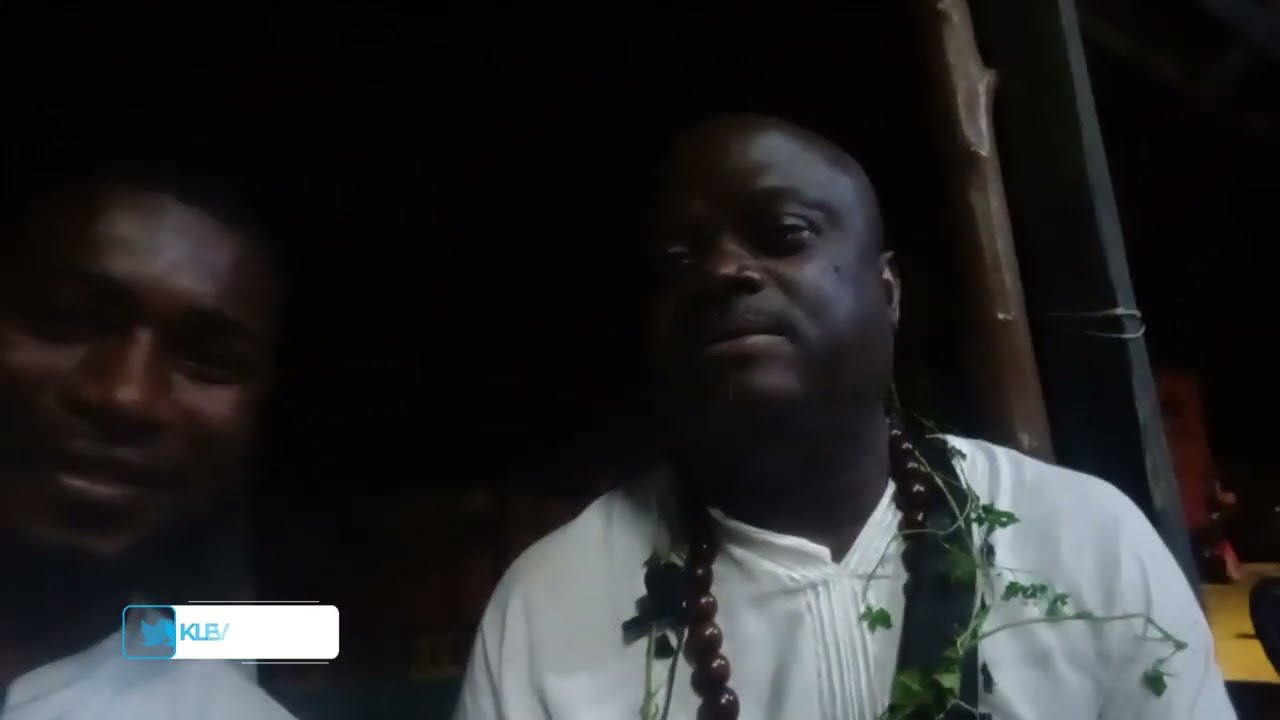In this image, two men of African-American ancestry stand side-by-side, possibly taking a selfie. Both are dressed in white shirts, which might be traditional African attire. The man on the right wears a necklace made of brown beads, along with a vine-like green herb around his neck and a black strap over his shoulder. The man on the left, who appears to be taking the photograph, leans towards his companion. The background is very dark, suggesting it may have been taken at night. They are positioned under a porch with two wooden poles on the right and a yellow, tan-hued floor beneath them. In the distance, a large red chair resembling a throne is visible. A white logo featuring the blue letters "KLB" can be seen in the bottom left corner of the image.